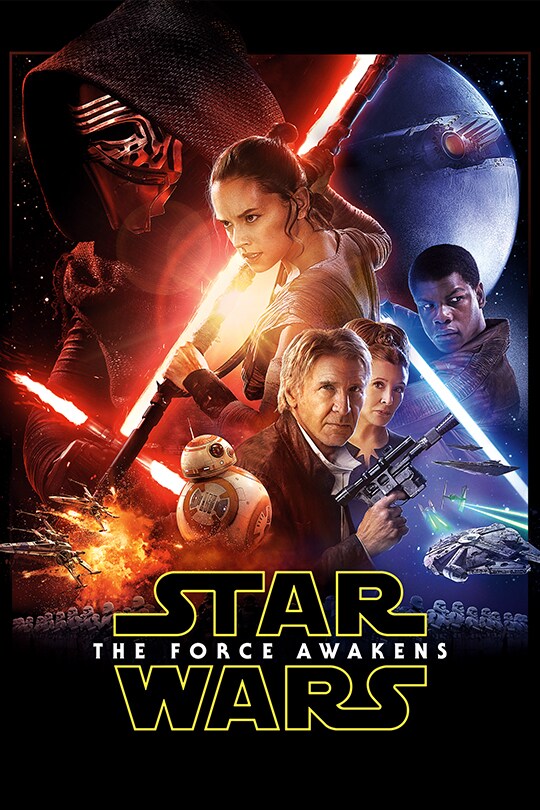This movie poster for "Star Wars: The Force Awakens" features an iconic collage of the main characters against a black backdrop, capturing the essence of the Star Wars saga. Positioned prominently in the top left, Kylo Ren, masked and hooded in black with a red crossguard lightsaber, looks menacing. At the center stands Rey, her hair in a bun, firmly gripping her staff and gazing left. Surrounding her, we see Han Solo (Harrison Ford) holding his pistol and Leia Organa, both looking directly into the camera. The character Finn, portrayed by John Boyega, is on the far right, framed by the chaos of battle. Below Finn, the Millennium Falcon rockets away from a fiery explosion, pursued by TIE fighters and accompanied by two X-wing fighters. Near Han Solo’s right shoulder, the spherical droid BB-8, colored in white and orange, is also seen escaping the explosion. The backdrop includes images of stormtroopers and the ominous Death Star looming in the top right. At the bottom of the poster, the familiar Star Wars logo sits with "The Force Awakens" vertically between "Star" and "Wars," perfectly encapsulating the epic's adventurous spirit.